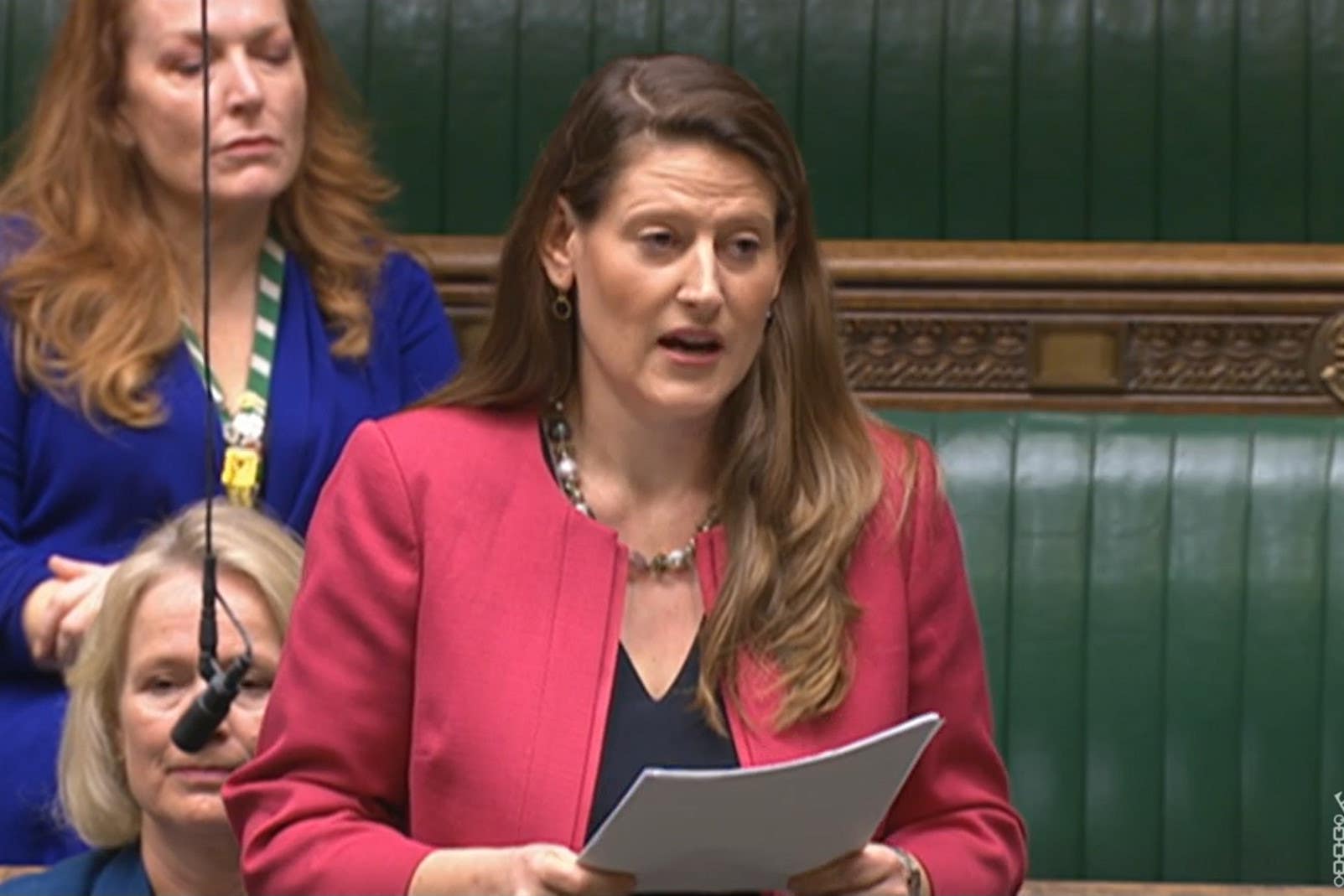The image captures a formal setting, possibly a courtroom or government chamber, marked by green walls extending down to a brown, ornately detailed wooden trim that may serve as decor or seating. Three women are present. The woman in the forefront, a Caucasian female with long, straight, brown hair parted to the right, is speaking and holds a stack of white papers. She is dressed in a red jacket over a black V-neck shirt, and her ensemble is accessorized with a prominent gold, white, and gray necklace, as well as small hoop earrings. A microphone hangs down from above, positioned near her. 

Behind her, seated on green leather benches, is a blonde woman who gazes off to the side, appearing attentive. She is positioned near the microphone, which suggests she may speak next. To her left, standing further back, is a woman with closed eyes and reddish hair, either caught mid-blink or in a candid, unaware moment. This third woman is dressed in a light navy blue sweater or dress and wears a green and white lanyard around her neck holding keys. The overall scene conveys a serious and focused atmosphere.